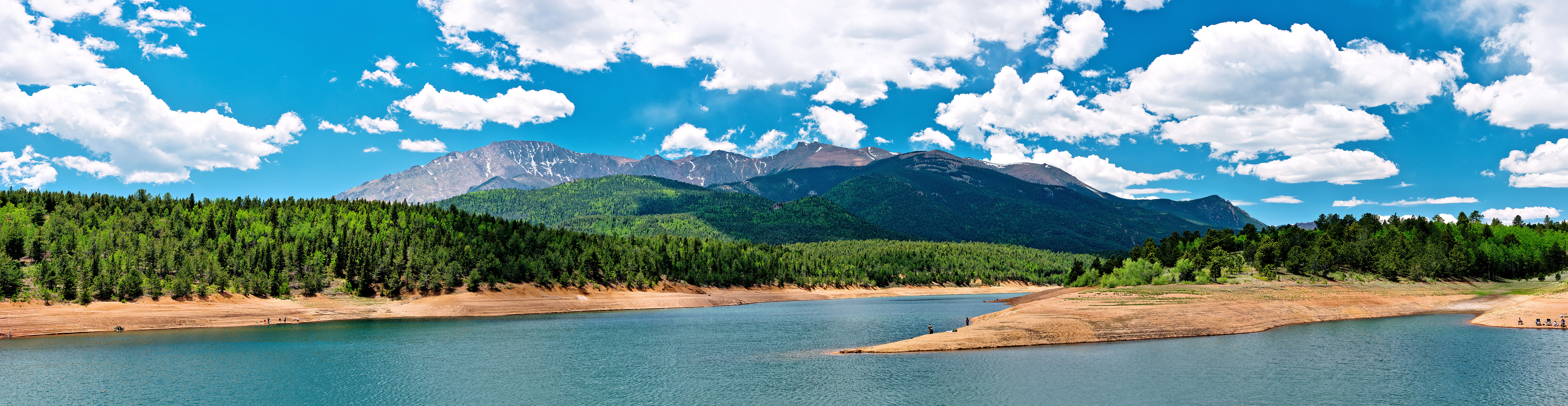The image captures a tranquil lake in a super landscape orientation, expansive left to right and relatively short in height. The crystalline water stretches from the foreground to the horizon, meeting a jutting piece of land devoid of vegetation, suggesting it might be sand or bare soil. Beyond the shoreline, a dense cluster of trees, possibly conifers, frames the scene. In the background, towering mountains rise majestically, their peaks potentially dusted with snow. The sky above is a vivid blue, dotted with numerous fluffy white clouds, adding to the serene and majestic ambiance of the landscape.